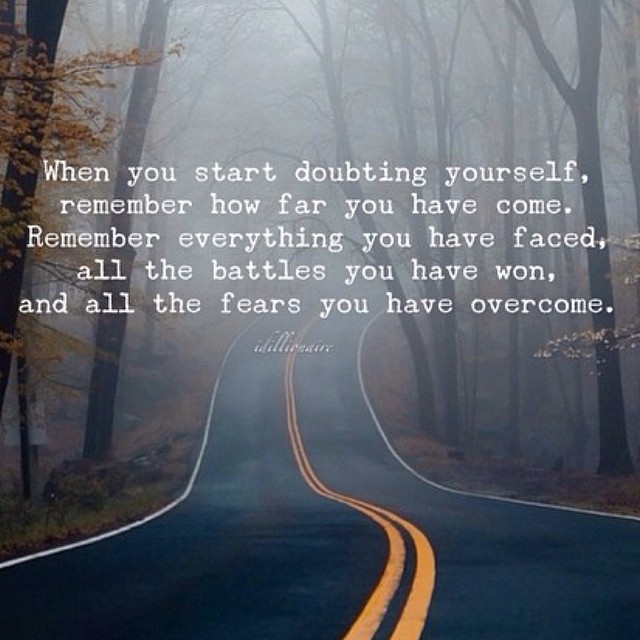The image features a winding, paved country road with two solid yellow lines running down the center. Flanked by tall, thin trees adorned with orange and yellow leaves, the road appears shrouded in dense, misty fog that conveys a sense of quiet solitude. The season suggests fall, with many dead leaves scattered on the ground. Above the road, white text overlays the scene, offering an inspirational message: "When you start doubting yourself, remember how far you have come. Remember everything you have faced, all the battles you have won, and all the fears you have overcome." The photo, captured in a vertical rectangular format, shows the road curving off to the right in the distance, bathed in diffused daylight.